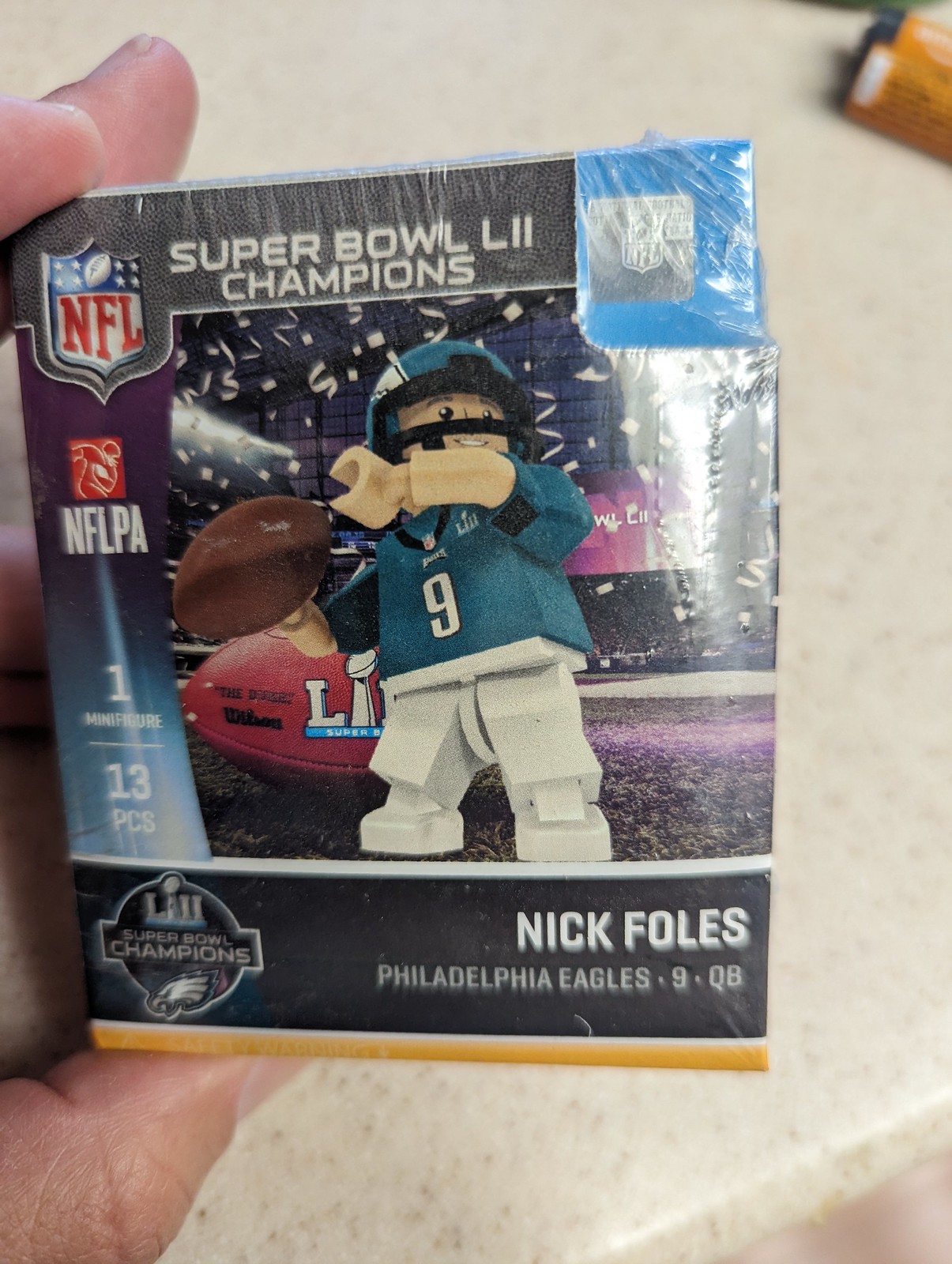The image depicts a hand holding a small box featuring a Nick Foles bobblehead styled as a Lego-like figurine. The packaging prominently declares "Super Bowl LII Champions" at the top, along with an NFL logo displaying the iconic red letters, white background, and blue border with stars and a football. The figurine, dressed in a turquoise Philadelphia Eagles jersey, white pants, and a helmet, is posed with a football in its right hand, poised as if ready to throw. The background of the box showcases a vibrant scene with confetti and purple lighting, enhancing the celebratory Super Bowl theme. The black sections at the top and bottom of the box include text that reads "Nick Foles, Philadelphia Eagles, #9 QB." The hand holding the box is positioned over a speckled, cream-colored surface, with the box's size indicated by the visibility of the fingertips.